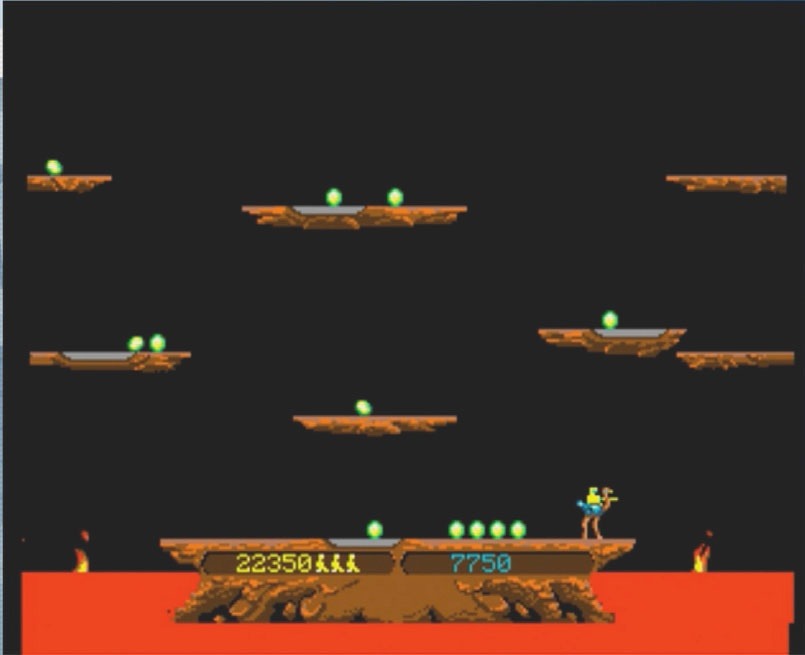A vivid scene from a video game captures a character standing poised on a narrow ledge surrounded by a sea of fiery orange-red. The ledge is perched precariously above what appears to be a pit filled with molten lava, with occasional flames licking upwards. On the ledge, the character is preparing to jump towards several floating platforms suspended in mid-air. These platforms are adorned with clusters of bright yellow orbs encircled by blue, which are scattered like diamonds across the space. The objective seems to involve skillfully navigating through the air, leaping from platform to platform to collect more of these glowing orbs, while avoiding the perilous fire hazard below.